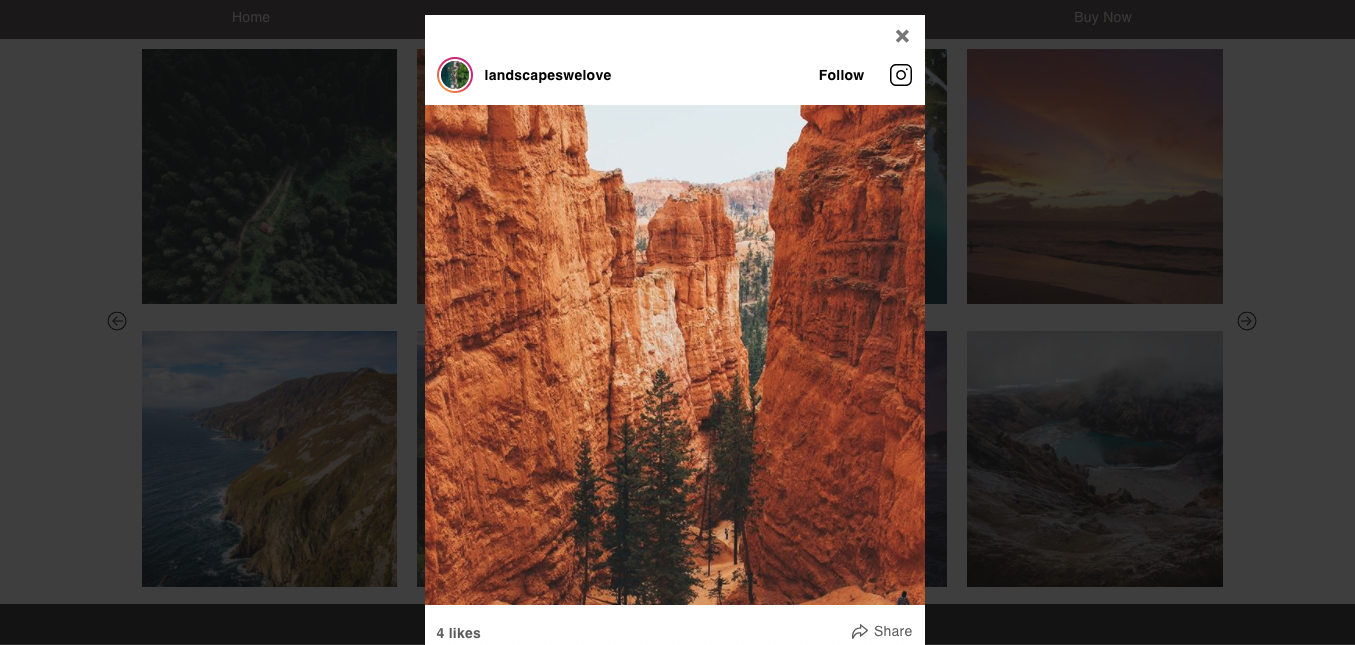The image depicts a breathtaking view reminiscent of the Grand Canyon, with towering red rock formations flanking either side of a narrow, high-walled canyon. The striated rock layers are prominently visible, showcasing a rugged, textured landscape. Nestled within the valley between the rock faces are tall, slender evergreens, resembling pencil-shaped Christmas trees, interspersed amidst the imposing stone. The background reveals additional evergreen trees and the faint outlines of distant mountains.

At the base of the image, an interactive feature indicates "four likes" and options to share. The left side of the image includes grayed-out, shadowy mountain figures, adding to the depth but lacking clear details. On the right side, a vivid image suggests a scenic sunset possibly over water, complemented by another smaller, slightly obscured depiction of rocky terrain and water below.

Prominently positioned in the middle is a banner labeled "Landscapes We Love," adorned with an icon featuring trees and land. Users can engage with or follow the account as indicated by a box with a circle and an "X" above it, integrating social media elements into the visual experience.